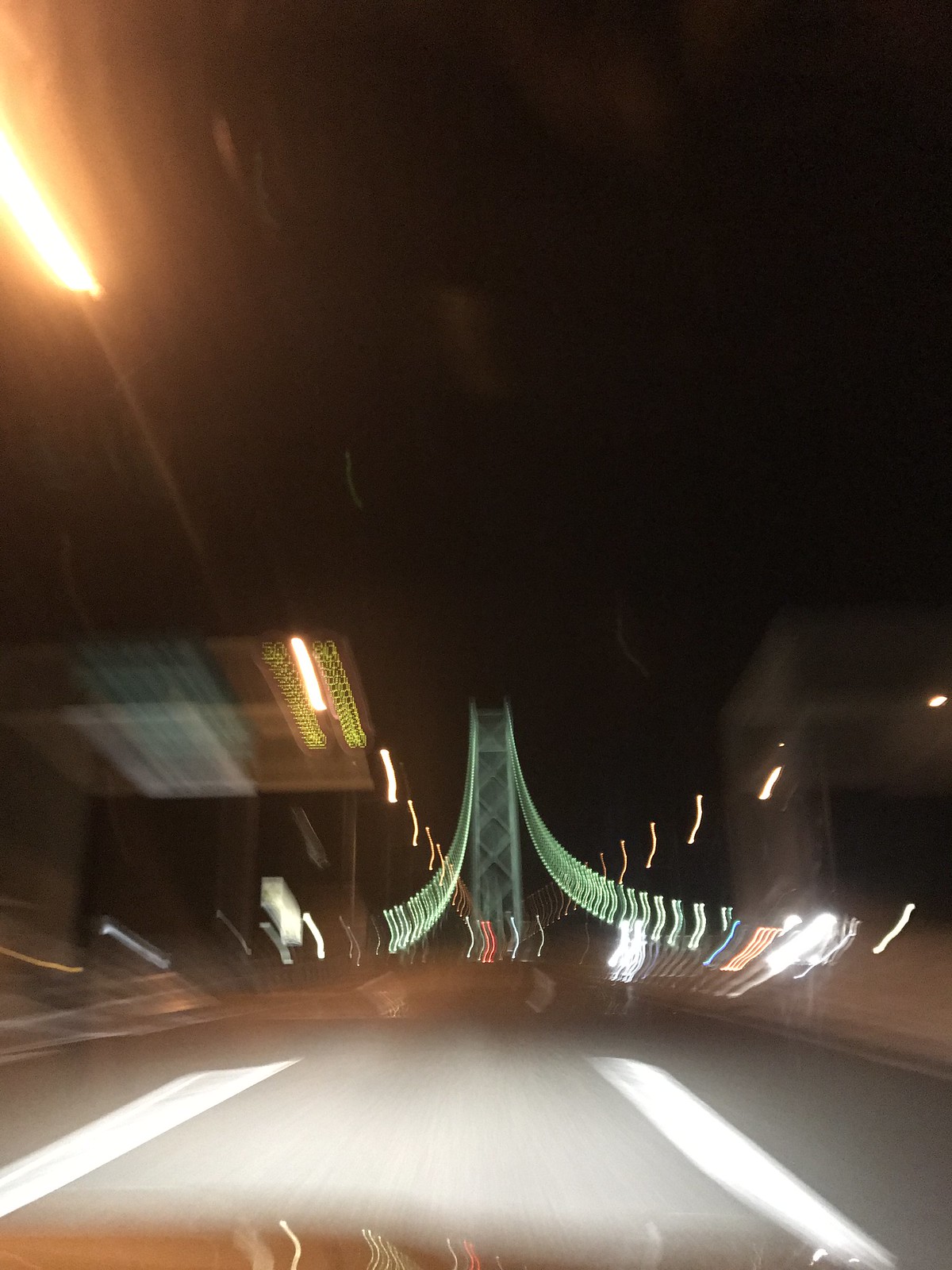A night-time street scene captured from a moving vehicle. In the foreground, the road is marked with two clearly defined lane lines, guiding the path ahead. Above, a bridge looms in the distance, its structure illuminated with a near-white light, while its sides exhibit a faint greenish tint. The motion of the vehicle is evident from the streaks of light trailing from the street lamps. To the left, an overhanging structure resembling a roof hovers above the scene, contributing to the urban landscape. On the topmost part of the image, a prominent light is visible, with another coming into view further ahead. To the right, a cemented structure with a distinct front rises, its top part contrasting against the dark night sky, which forms the backdrop for this dynamic and vibrant roadway capture.